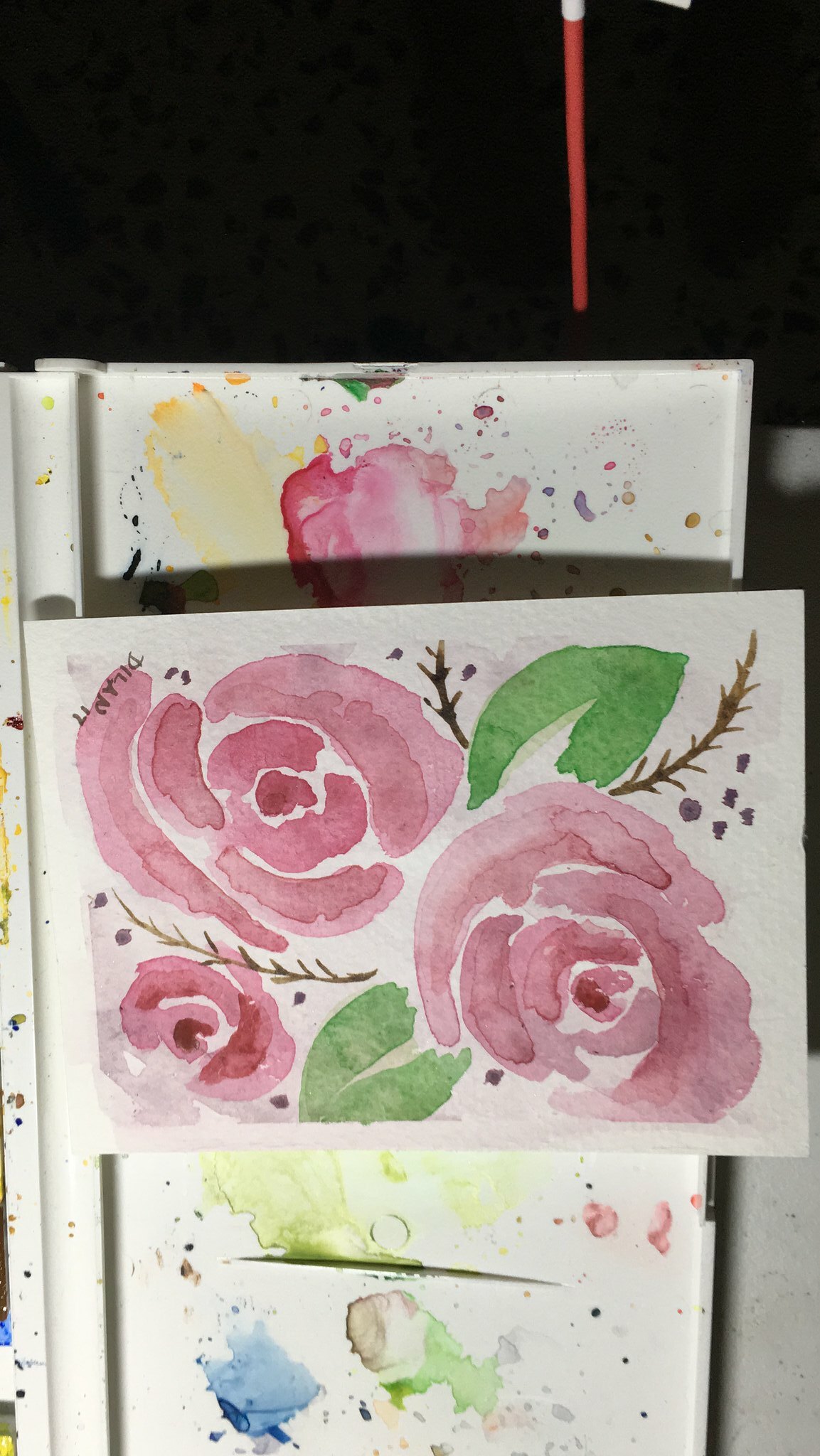This image captures an artist's watercolor setup in beautiful detail. At the center of the composition lies a small, vertically-oriented white canvas sheet, featuring a delicate watercolor painting. Prominently displayed on this canvas are three vividly painted pink roses, accentuated by two lush green leaves and three elegant brown branches. The roses are interspersed with subtle purple and blue splotches, hinting at a playful background. The lower left-hand corner of this canvas showcases an unreadable signature. 

Surrounding this central piece, a plastic easel or backdrop is heavily dotted with splashes of various watercolor pigments—orange, yellow, blue, green, and more—hinting at the artist's vibrant palette. Behind the artwork, the background fades into darkness, except for a striking red cable leading upwards. This setting gives the entire scene a sense of depth and artistic chaos, reflecting the creative process at work.